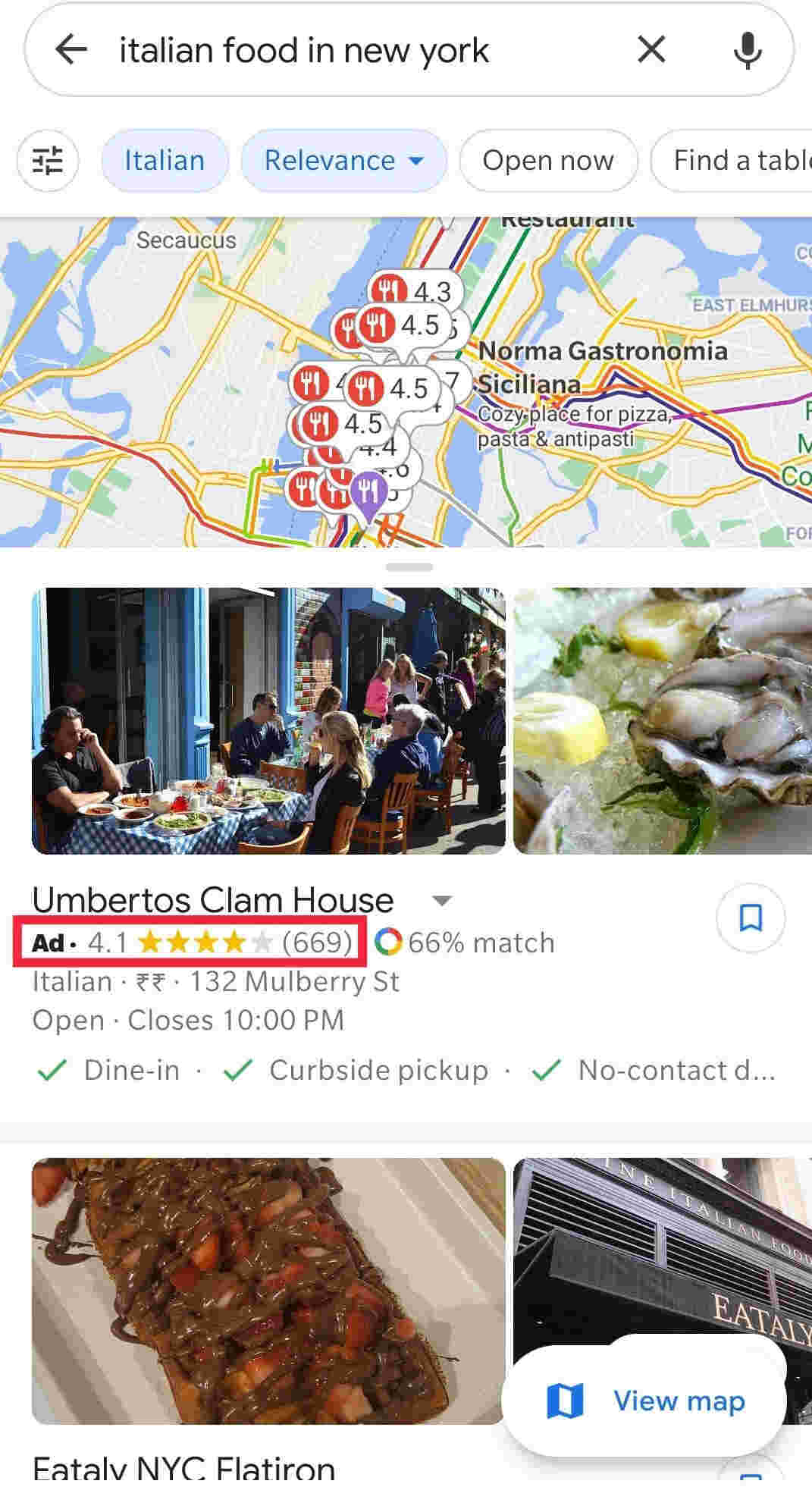This image captures a screenshot of a Google search query for "Italian food in New York," viewed on a mobile device. The portrait-oriented screen primarily against a white backdrop features a horizontal search bar at the top with the query "Italian food in New York," flanked by icons for a back arrow, an 'X', and a microphone. Directly beneath the search bar are filter options, including a blue bubble labeled "Italian," another blue bubble labeled "Relevance" with a dropdown menu, and two white bubbles labeled "Open now" and "Find table."

The middle section of the screenshot displays a landscape-oriented map showcasing various restaurant locations, each marked with ratings. Below the map is a split image: on the left, people are shown dining al fresco at a restaurant, and on the right, a dish featuring clams and lemon wedges. 

The bottom section highlights a specific restaurant, "Umberto's Clam House." It includes a header with the restaurant’s name, marked as an ad, with a star rating of 4.1 out of 5 based on 669 reviews. A label indicates that the search result has a "66% match." Beneath this, it states the restaurant’s cuisine ("Italian"), address (123 Mulberry Street), and operating hours (open, closes 10 p.m.). Finally, it lists the available services: dine-in, curbside pickup, and non-contact delivery.